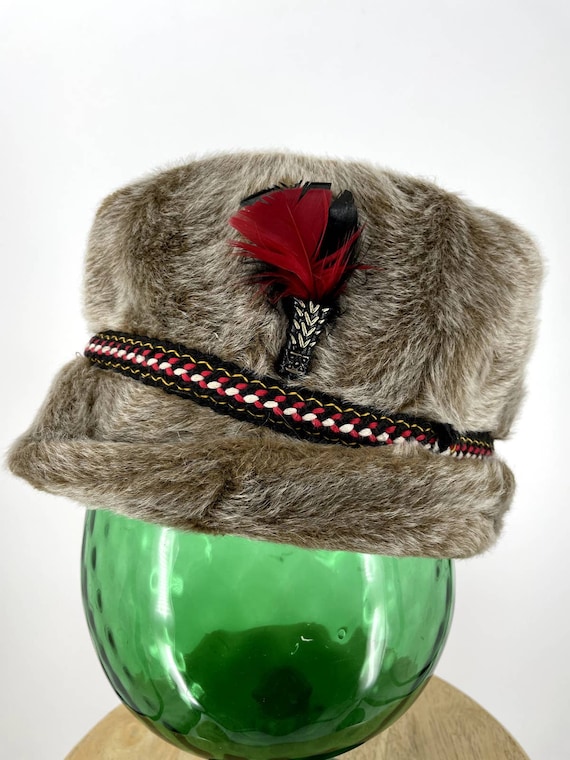This image is a carefully staged artistic still life photograph capturing a vintage, fur-like hat. The hat, with its textured, wispy fur resembling that of a rabbit, shows a mix of white, brown, and gray hues. It features a distinctive headband in red, black, and white, accented with a golden trim. A pair of feathers, one red and one black, elegantly protrudes from the side of the band. Perched atop a green, nubby-patterned glass sphere, this glass object evokes the suggestion of a human head. The entire arrangement rests upon a small, oval wooden table, set against a pristine white background. The overall composition emphasizes the contrast and interplay of textures and colors, highlighting the vintage charm and intricate detailing of the hat.